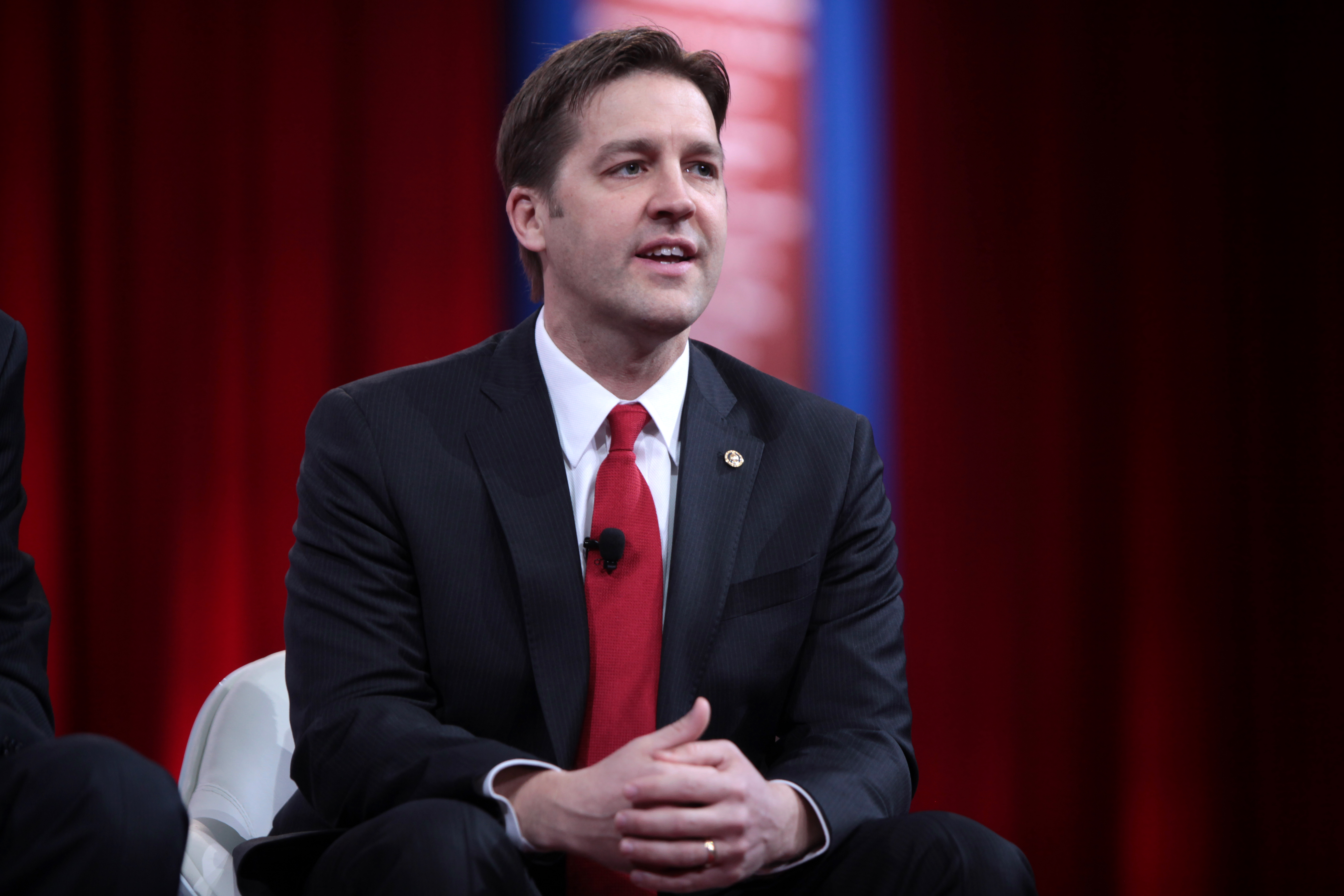The photograph captures a clean-shaven, white gentleman in his 40s, dressed in a suit consisting of a black jacket, white collared shirt, and red tie, with a notable gold pin on his right lapel. He has short brown hair neatly parted. Sitting in a white chair, his hands are interlocked, highlighting his gold wedding ring. A microphone is clipped onto his tie, suggesting he is in mid-speech, with his mouth open and eyes focused slightly to the right. The backdrop features a rich red curtain, and there is a hint of a red, white, and blue sign blurred in the background. The photo appears slightly wider than it is tall, giving a full view of him seated with part of another person cut off to the left. The scene suggests a public speaking event or political gathering.